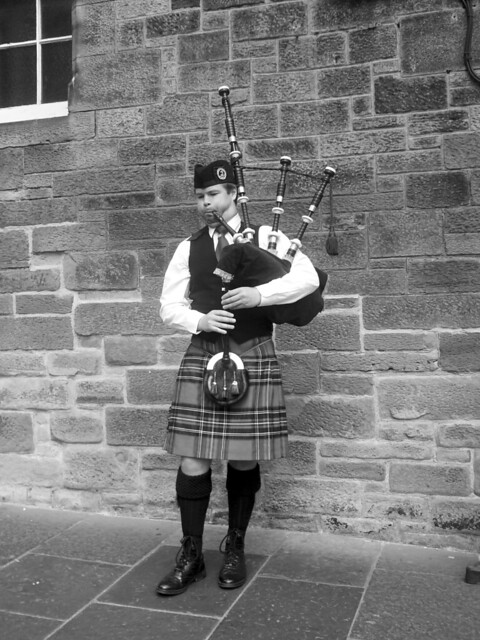This black and white photograph captures a man playing the bagpipes on a cobblestone street, standing in front of a brick wall with a window on the top left-hand side. The man, the main focus of the image, is donning a traditional outfit, including a black hat, a black vest over a white long-sleeved dress shirt, and a plaid kilt, which appears in shades of gray due to the monochrome nature of the photo. His attire is completed with high knee socks and black laced-up shoes. As he plays, his cheeks are visibly puffed up. The bagpipes, with four protruding pipes, are also black, matching his hat and vest. This artistic photo emphasizes both the traditional elements of his clothing and the historical ambiance of the cobblestone street and brick building.